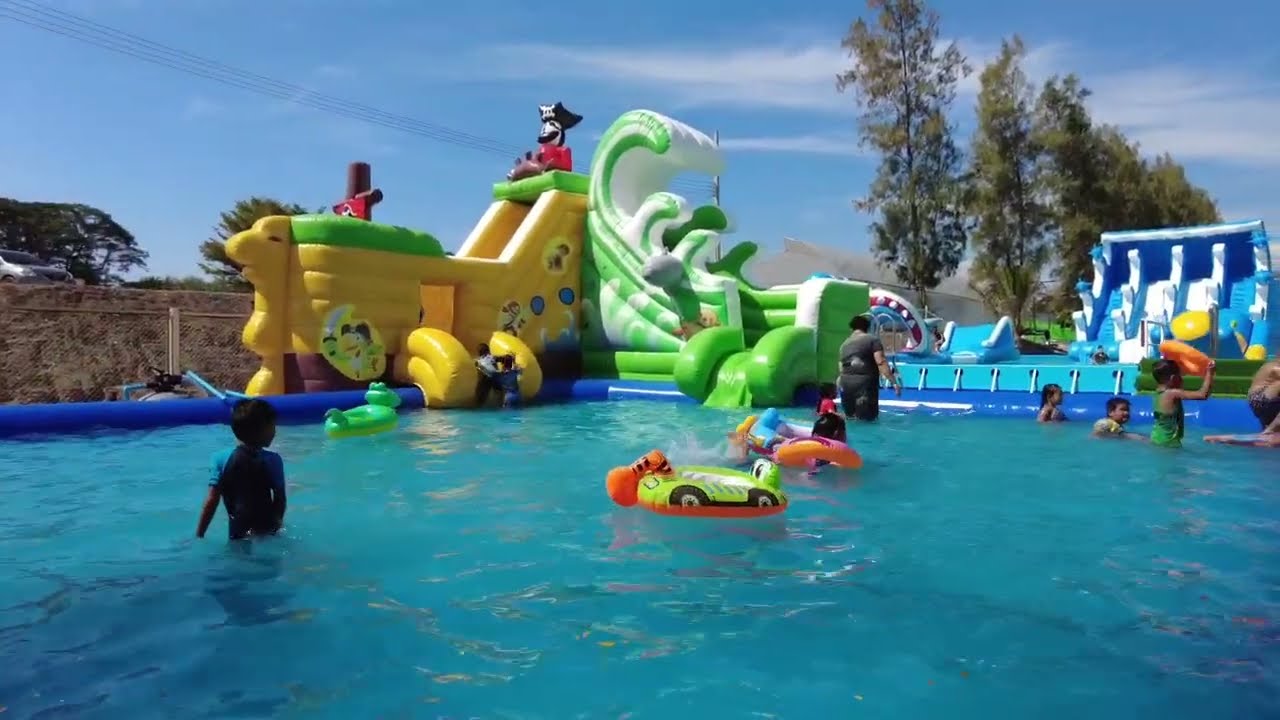The photograph captures a vibrant outdoor water play area on a bright, sunny day with a blue sky streaked by a few white clouds. Dominating the scene is a large, rectangular swimming pool, encircled by several colorful inflatable structures, including a yellow pirate ship-themed slide complete with a pirate dressed in a black hat and red shirt at the helm, and a green-and-white wave-shaped slide. Perpendicular to these, another inflatable structure features blue and white lanes for sliding. In the pool, which appears shallow enough for toddlers, are about six children and a few adults supervising. Scattered across the water are three animal-shaped, colorful floating inner tubes. Surrounding the pool area are tall trees, and in the right background, another pool area with additional inflatables can be seen. The entire scene exudes a lively and playful atmosphere, with everyone clearly enjoying the sunny day.